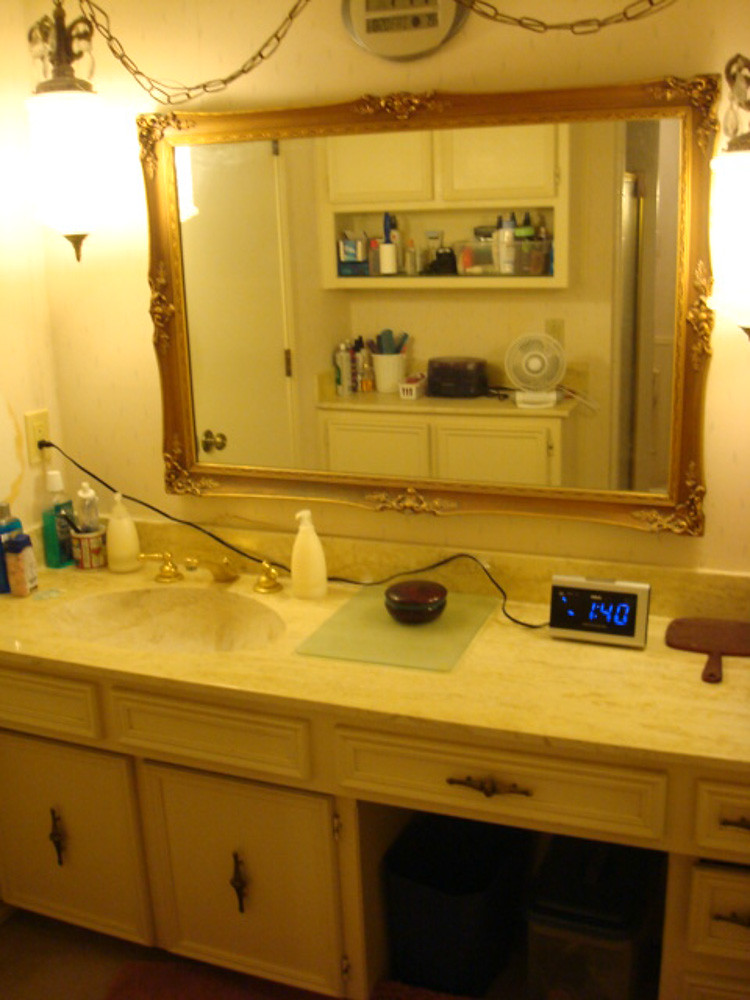This image captures a tastefully styled bathroom, viewed from a right angle with a subtle yellow tint. The sink, situated on the right side, is crafted from elegant marble and adorned with gold-handled faucets. On either side of the sink, two white bottles are placed, flanked by a toothbrush holder with a toothbrush, mouthwash, toothpaste, and what appears to be some medicine.

An electrical outlet and plug feature prominently, with a cord stretching across the sink to connect to a gray alarm clock displaying "1:40" in blue digits. Beneath the sink area, a mat with a bowl adds a functional touch to the space.

Dominating the wall is a large, gold-framed mirror, while its grandeur is accentuated by lights on either side, suspended by delicate chains. The right side of the bathroom hosts a trash can and a storage box, completing the room’s organized yet sophisticated aesthetic.